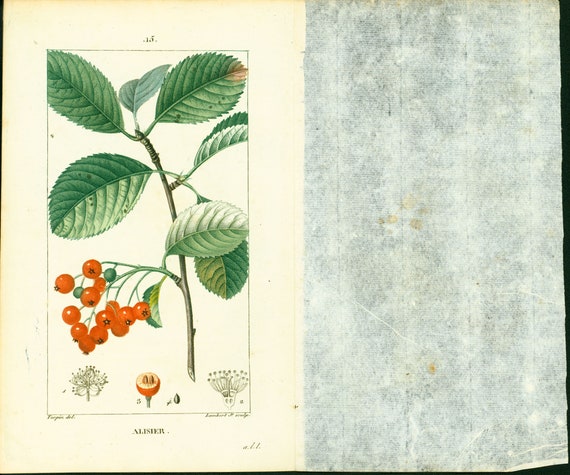This image appears to be a detailed page out of a book or an informational sheet, featuring a botanical illustration of a plant branch. The plant has a stem adorned with numerous large, green, oval-shaped leaves. One section of the stem showcases a cluster of small, round, orange berries, with a couple still green, indicating they aren't yet ripe. At the bottom of the page, there is a detailed illustration of one of these berries cut in half, revealing that it contains two seeds. Additionally, there is a depiction of a berry or flower blossom. The background on the right side of the image is grayish-blue, possibly indicating a textured paper or a wall. The bottom text appears to spell out a name, possibly "ALISHER" or "LALISIER."